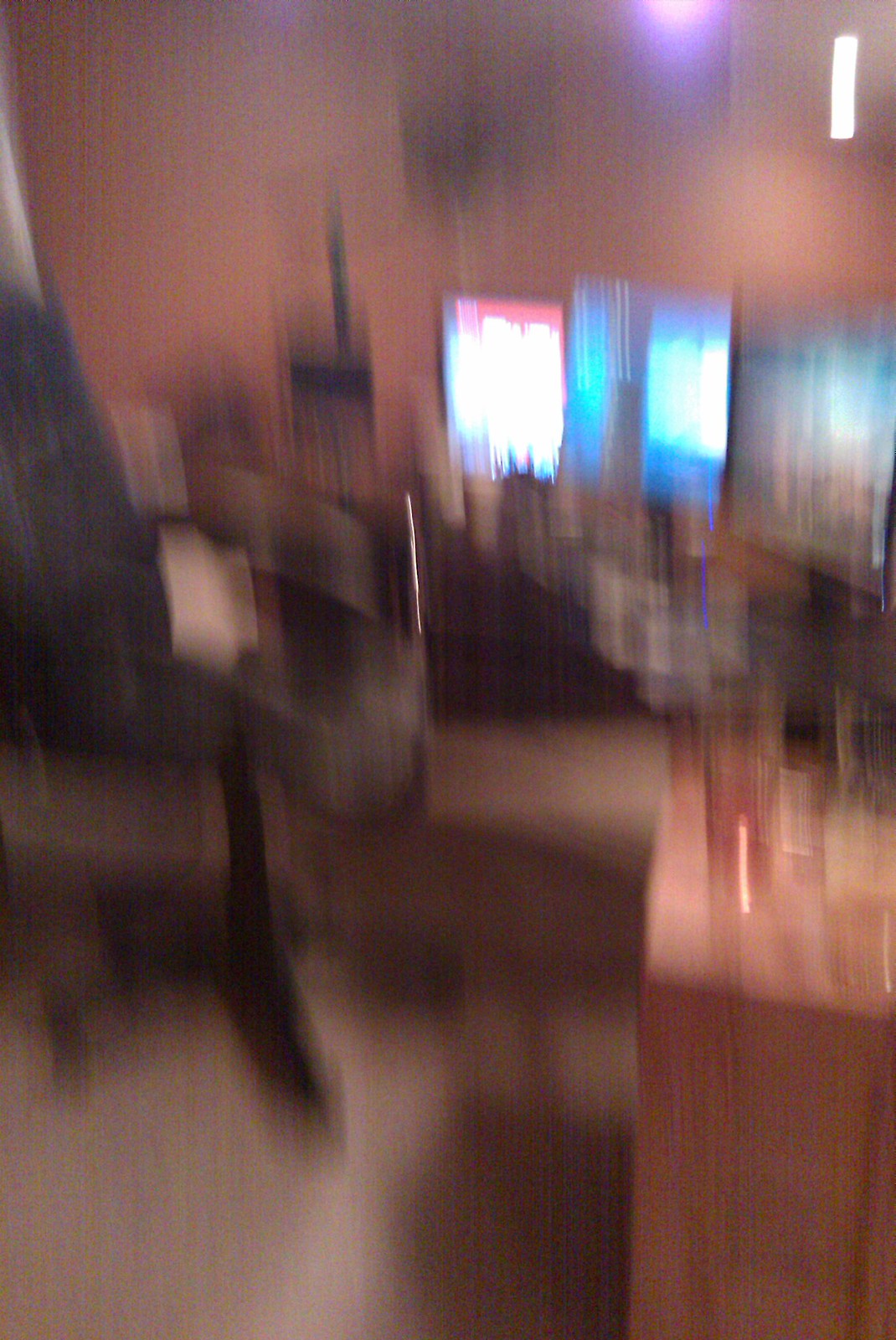The image depicts a blurry photograph of what appears to be an office setting. Dominating the room is a likely L-shaped or wraparound brown desk, accompanied by a shiny object, possibly a cup, placed on top. Positioned in front of this desk is a black computer chair. Visible within the somewhat shaky shot are three illuminated screens, each emitting different levels of light—a brightly lit one on the left, a blue-reflecting screen in the middle, and a dimly lit one on the right. The walls in the background showcase a brownish hue, with potentially some black elements toward the bottom. The flooring appears to be a light tan or pinkish-grey carpet that absorbs various shadows. Additionally, there could be a black object resembling a router situated in the back, contributing to the overall office ambiance captured in this photograph.